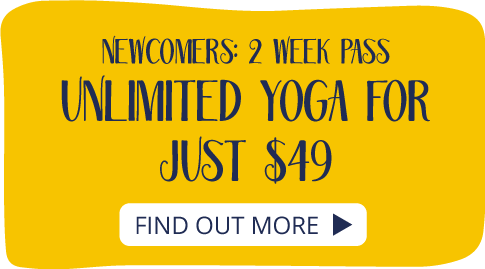The image is a graphical illustration, likely designed for use as an advertisement on a website or mobile app. The layout is landscape-oriented with wavy edges, creating a visually engaging frame. The primary background is a solid yellow rectangle, which contrasts with the black text and a prominent white button.

The text, which is all in uppercase, is in a decorative sans-serif font with elongated letters and slight curlicues, adding an elegant and modern touch. It reads: "Newcomers: Two-Week Pass Unlimited Yoga for Just $49." 

Centered near the bottom of the yellow background, there's a stark white button featuring additional black text that urges the viewer to "Find Out More," accompanied by a right-pointing black arrow, encouraging user interaction. The overall design is minimalistic, focusing on the promotional offer without any extraneous details about the entity behind the advertisement, which might be a yoga studio or gym.